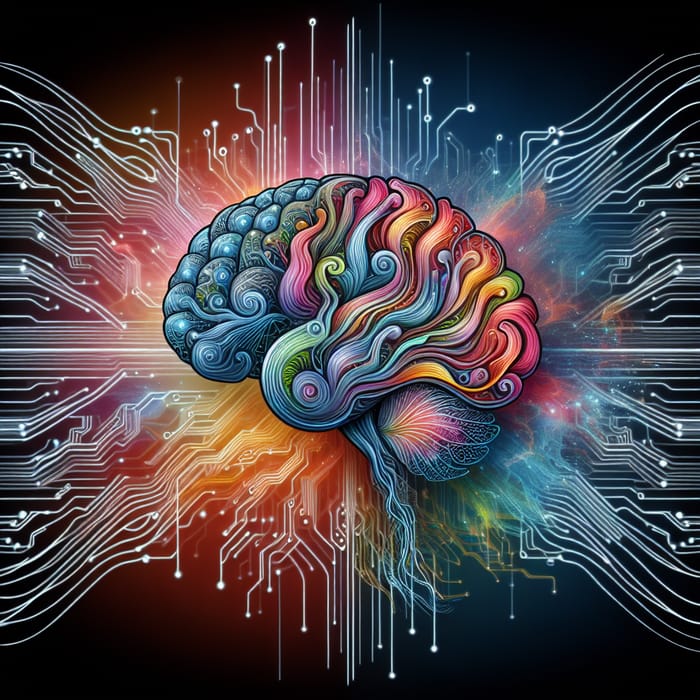This vibrant image resembles a dynamic painting, characterized by a rich array of colors. The backdrop is a deep, almost velvety black, scattered with intricate white lines shooting in various directions, creating a sense of movement and depth. Dominating the center is a complex, brain-like shape bursting with color. The left side of this central form is predominantly blue, subtly blended with hints of green. As we move towards the middle, a vibrant cacophony of pinks, purples, greens, oranges, and yellows takes over, cascading downward in strands that evoke the fluid, flowing nature of hair or the delicate tentacles of a jellyfish. Adding to the intricate design, feather-like appendages extend from the back, enhancing the ethereal and organic quality of the piece.